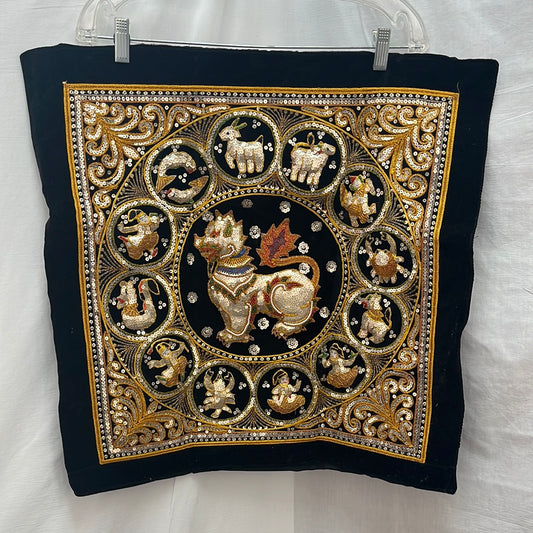This image showcases a black square piece of fabric, possibly a pillow cover, suspended by a hanger with metal clips, reminiscent of a pants hanger. The fabric is set against a white linen background, emphasizing its intricate details. 

At the center of this black fabric is a gold square surrounded by an elaborate embroidery pattern. This pattern includes ornate borders, with the corners adorned in a filigree design. Encircling the gold square is a larger circle, which intersects each side of the square and contains 12 smaller circles. Each of these circles features detailed embroidery depicting various animals and figures, including a sheep or llama, a person, a crab, an elephant, a frog, and additional unspecified characters. These figures do not represent traditional zodiac symbols due to their variety and number.

At the core of this composition is a concentric black circle showcasing a prominent embroidered dragon, richly adorned with shiny jewels and silver sequins. The overall effect is one of opulence and intricate craftsmanship, with the sequins and embroidery adding depth and a touch of sparkle to the piece.